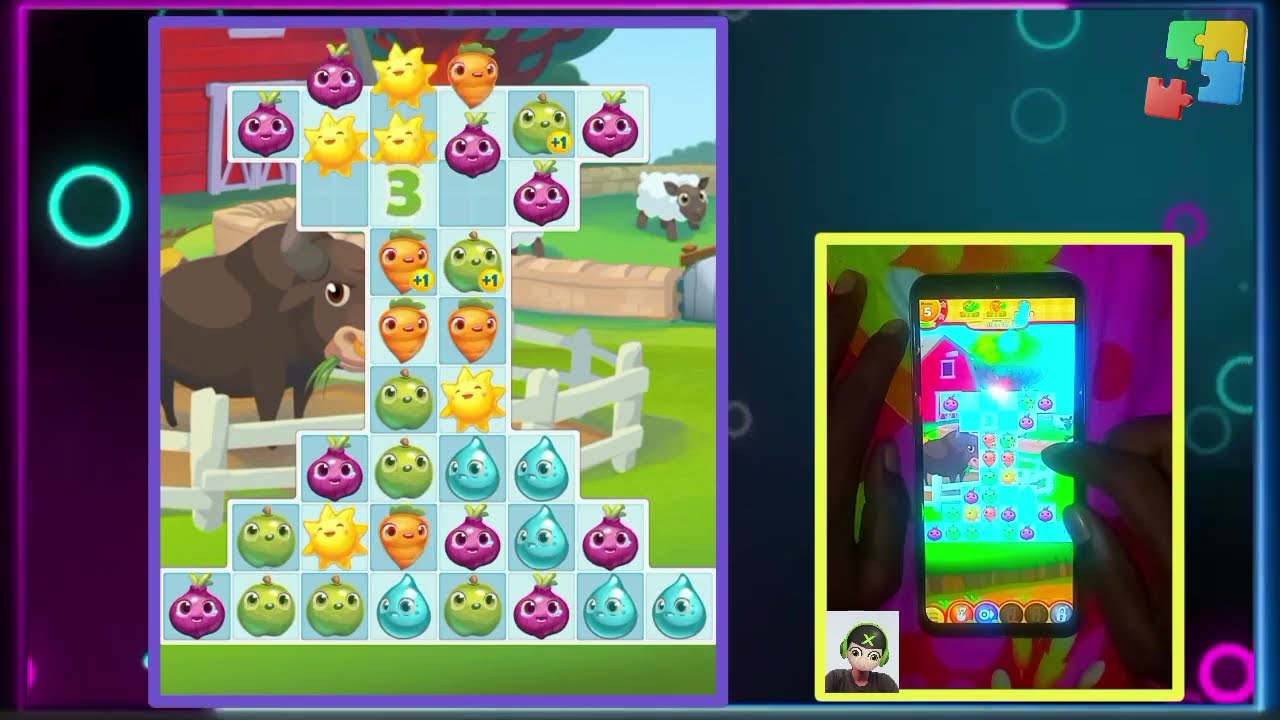This horizontal rectangular image, about six inches wide and three inches tall, appears to be a screenshot from a computer game. The background transitions from dark blue on the right to purple at the bottom left, eventually becoming black at the top left. In the upper right corner, there are a few puzzle pieces. The left side features an animal-themed background depicting a farm with a cow or bull on the left side and a lamb or sheep in the upper right-hand corner. These animals are separated by a small wall and encircled by a white fence. Additionally, a red barn is seen in the background behind the animals. The game itself is a match-three puzzle game played within a grid-like field composed of various colored icons, such as green apples, purple onions, blue water drops, golden suns, and orange carrots—all with cartoonish eyeballs.

On the right side of the image, there is a smaller rectangle outlined in neon yellow, showing a boy wearing green headphones in the lower left corner. Within this rectangle, the boy is holding an iPhone, demonstrating how the game is played on the device. The glowing screen illuminates his dark fingers as he interacts with the game, possibly while sitting on a blanket. The overall image has vivid neon outlines, adding to its vibrant and dynamic presentation.